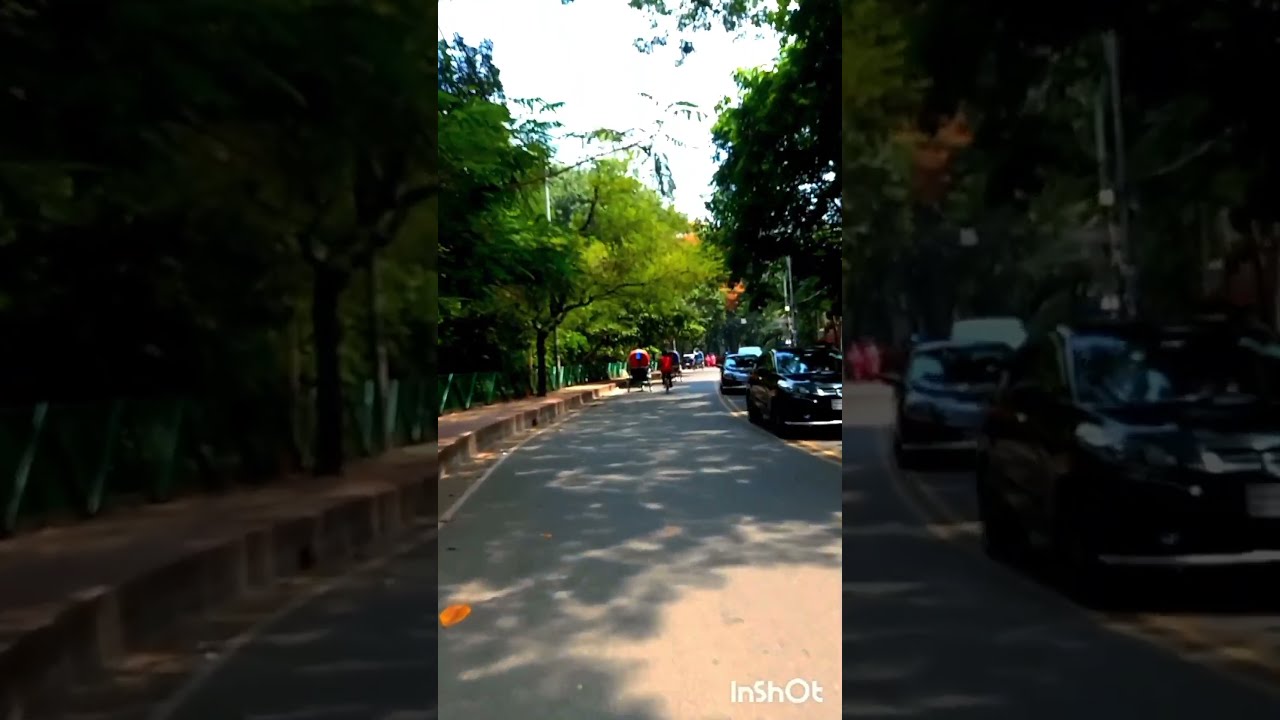The image centers on a photograph of a road with a distinctive layout, framed by enlarged and blurry versions of itself on the left and right thirds. The central photograph, taken in natural daylight, depicts a street where vehicles travel on the left side, suggesting it's set in a country with left-hand traffic. There is a reddish-colored concrete walkway on the left side of the road, bordered by a low wall or ledge. The road is flanked by trees on both sides, their branches and leaves partially overhanging the street.

To the right, cars are seen driving towards the observer, with some in the left lane of the road. In the distance, pedestrians or possibly cyclists are visible, moving along the left-hand lane. The bottom right corner of the main image is marked with the word "InShot." The blurred, zoomed-in sections on the left and right sides show close-up details of the sidewalks and cars, adding a dynamic frame to the central photograph. The overall composition suggests a bustling urban scene under natural light, with hints of daily traffic and pedestrian movement.